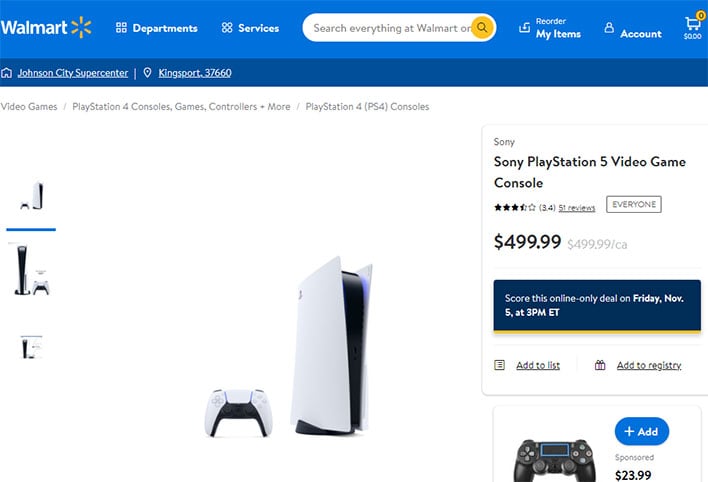This is a screenshot of Walmart's website, featuring a user interface designed primarily in blue with white text. At the top left corner, the Walmart logo is prominently displayed, accompanied by the yellow spindle icon resembling a flower. To the right of the logo, there are dropdown menus labeled 'Departments' and 'Services.' Below these menus lies the white search bar with a placeholder text reading, "Search everything at walmart.com," accompanied by a magnifying glass icon within an orange circle.

To the right of the search bar, options for 'Reorder My Items,' 'Account,' and the shopping cart are visible. The shopping cart icon shows an orange "0," indicating it's currently empty. The user's location is set to the Johnson City Supercenter in Kingsport with the ZIP code 37660.

The user is browsing the 'Video Game Consoles' section, specifically looking at 'PlayStation 4 consoles, games, controllers, and more.' Various images of PlayStation 4 products are displayed. On the right side of the screen, there's a listing for the Sony PlayStation 5 video game console, highlighted with a rating of 3.4 stars based on 51 reviews. The listed price for the PlayStation 5 is $499.